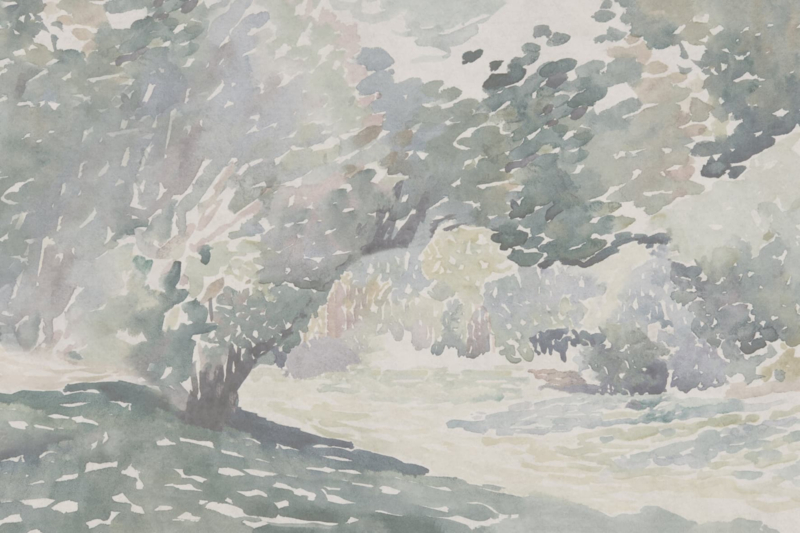This image features a calming and detailed watercolor painting dominated by light pastel shades of grays, taupes, pinks, and purples. The central focus is a tree standing on a small hill in the middle of a grove. The tree casts elongated shadows forward under the light gray sky. Surrounding the tree are smaller trees and bushes, with a winding pathway cutting through a meadow or grassy area. The painting is characterized by its splotchy texture, created with large dots of various sizes and a few brush strokes to define the tree trunk. The overall scene evokes a tranquil landscape, though its abstract and interpretive style could lead some to see varying elements such as erupting water or waves weaving through the foreground to the top right of the image.